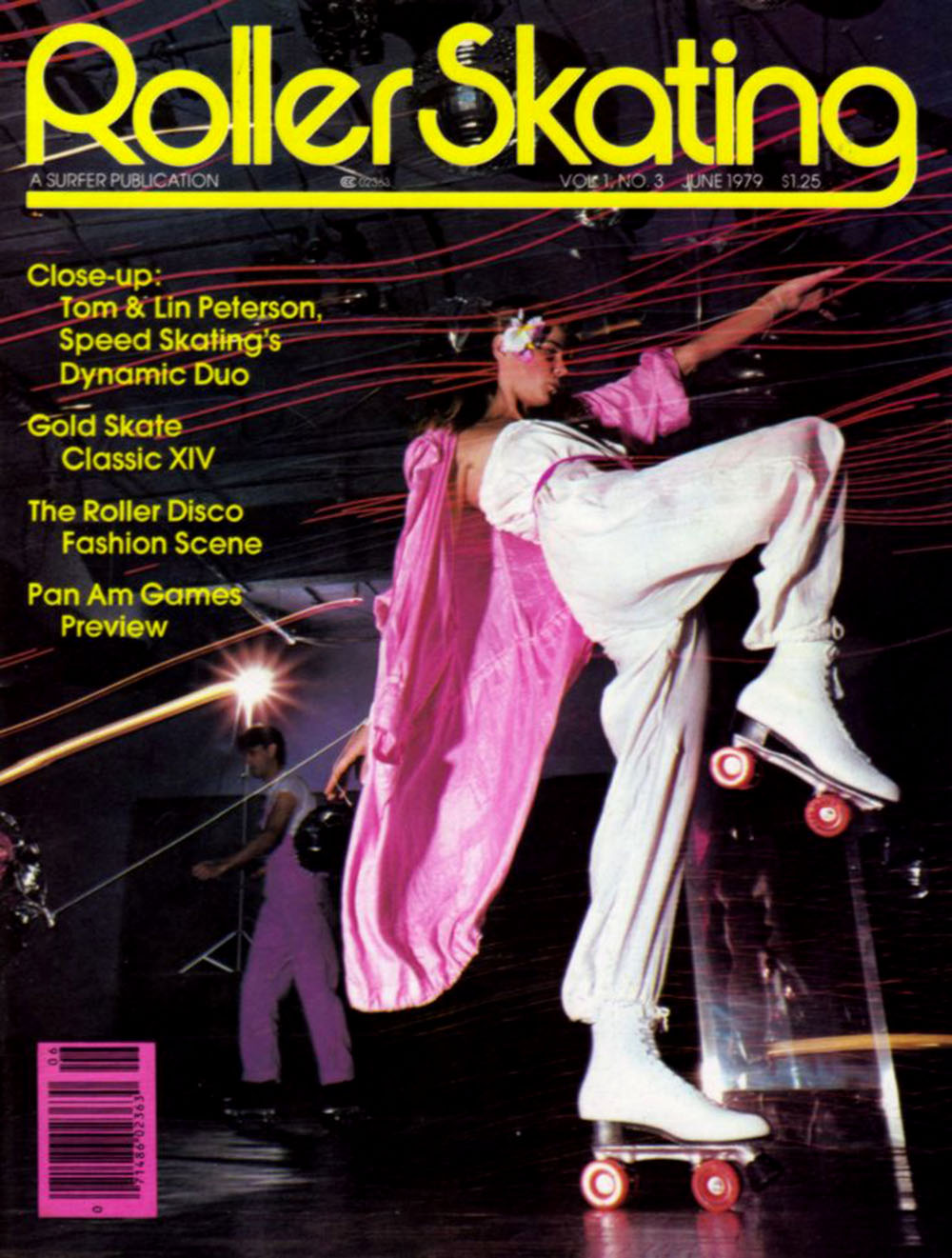The image is a vibrant magazine cover for "Roller Skating," prominently featuring the title in large yellow text. It highlights multiple articles, including "Close-Up: Tom and Lynn Peterson, Speed Skating's Dynamic Duo," "Gold Skate Classic XIV," "The Roller Disco Fashion Scene," and a "Pan Am Games Preview." At the forefront is a young, dark-haired woman possibly of Caucasian or Hawaiian descent. She is striking a dance pose with one foot up, roller skating on pink-wheeled white skates. She is outfitted in a stylish white strapless one-piece ensemble, paired with a pink covering, and adorned with a flower in her right ear. Behind her, likely her skate partner, stands a gentleman dressed in a matching white shirt and pink pants, both illuminated by a spotlight in an otherwise dark setting with wavy red lights. The detailed and dynamic composition effectively communicates the magazine's focus on the energetic world of roller skating.